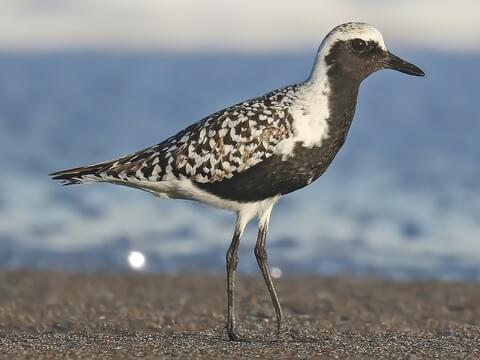A black and white bird, possibly a seagull, stands prominently at the center of the image, captured in a side view. It has a thin black beak and one visible beady eye, highlighted by a white cap on its head which extends down to its shoulders. The bird’s body features a speckled pattern of black, white, and brown, with some small brown flakes suggesting it's beginning to molt. Its front breast, the sides of its face, and part of its belly are black, while its underbelly and the area around its legs are white. The legs themselves are dark gray and appear very thin.

The bird stands on a pebbly beach near the shore, with the ground appearing soft and brown. In the background, the ocean extends into the horizon with sunlight reflecting off its surface, creating a glistening effect. The water looks relatively calm, and there are no other animals in sight. The entire scene is bathed in sunlight, adding a natural reflection on the ocean's surface. The bird seems to be casually strolling along the beach, not appearing to search for food or anything in particular.